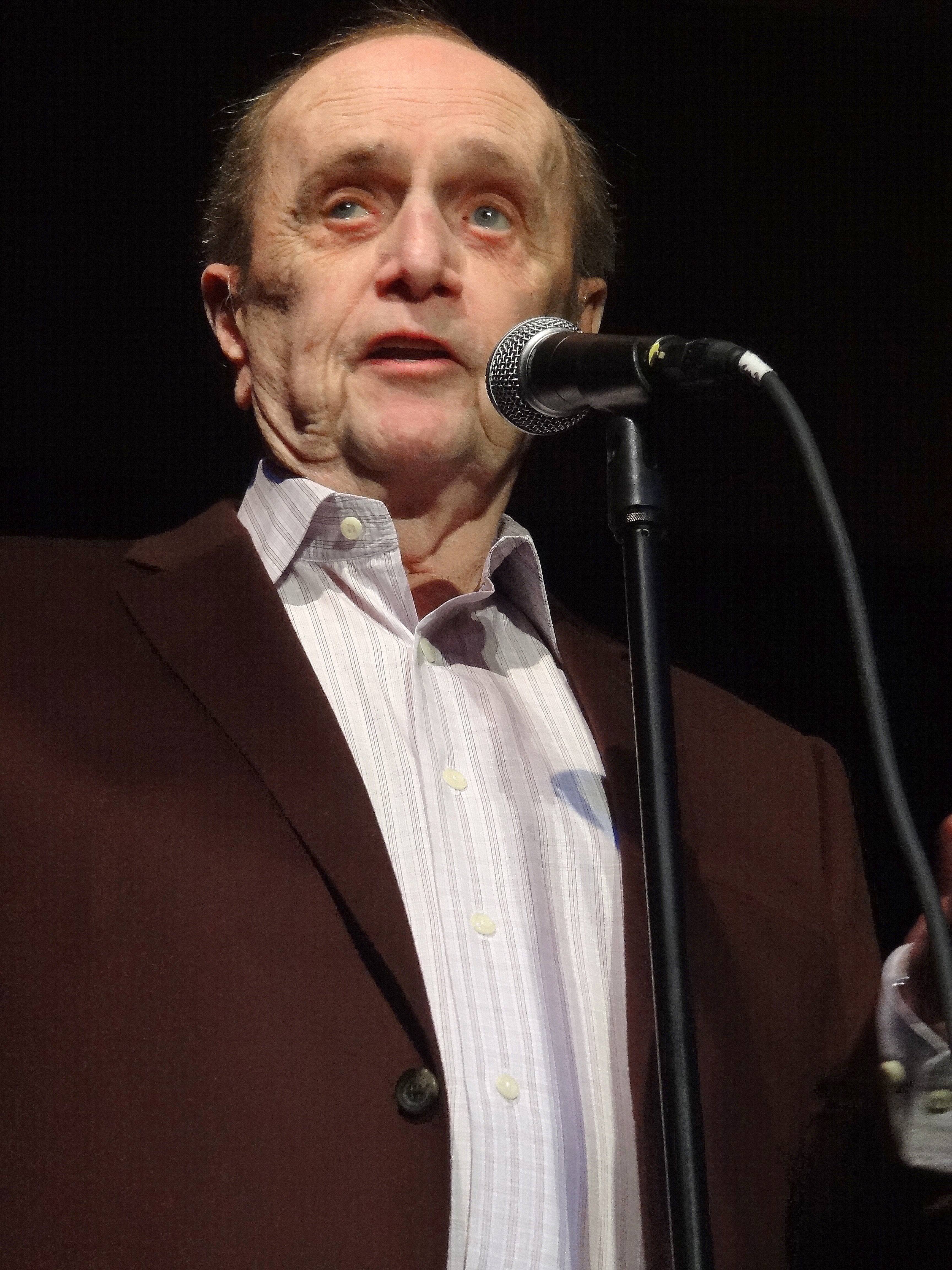This professionally taken photograph showcases the iconic actor and comedian Bob Newhart, positioned centrally and speaking into a silver and black microphone on a stand. Newhart, an older white male, appears engaged and is looking into the distance while addressing what seems to be a conference or comedy show audience. His attire includes a brown suit jacket with buttons over a light blue and white striped shirt, notably without a tie. His expression is serious, with his mouth slightly open as he speaks. The background is solid black, bringing focus entirely upon Newhart. The color palette of the image includes black, white, various shades of grey, silver, brown, light blue, peach, and beige. There are no textual elements or additional people in the picture, which emphasizes Newhart as the sole subject.